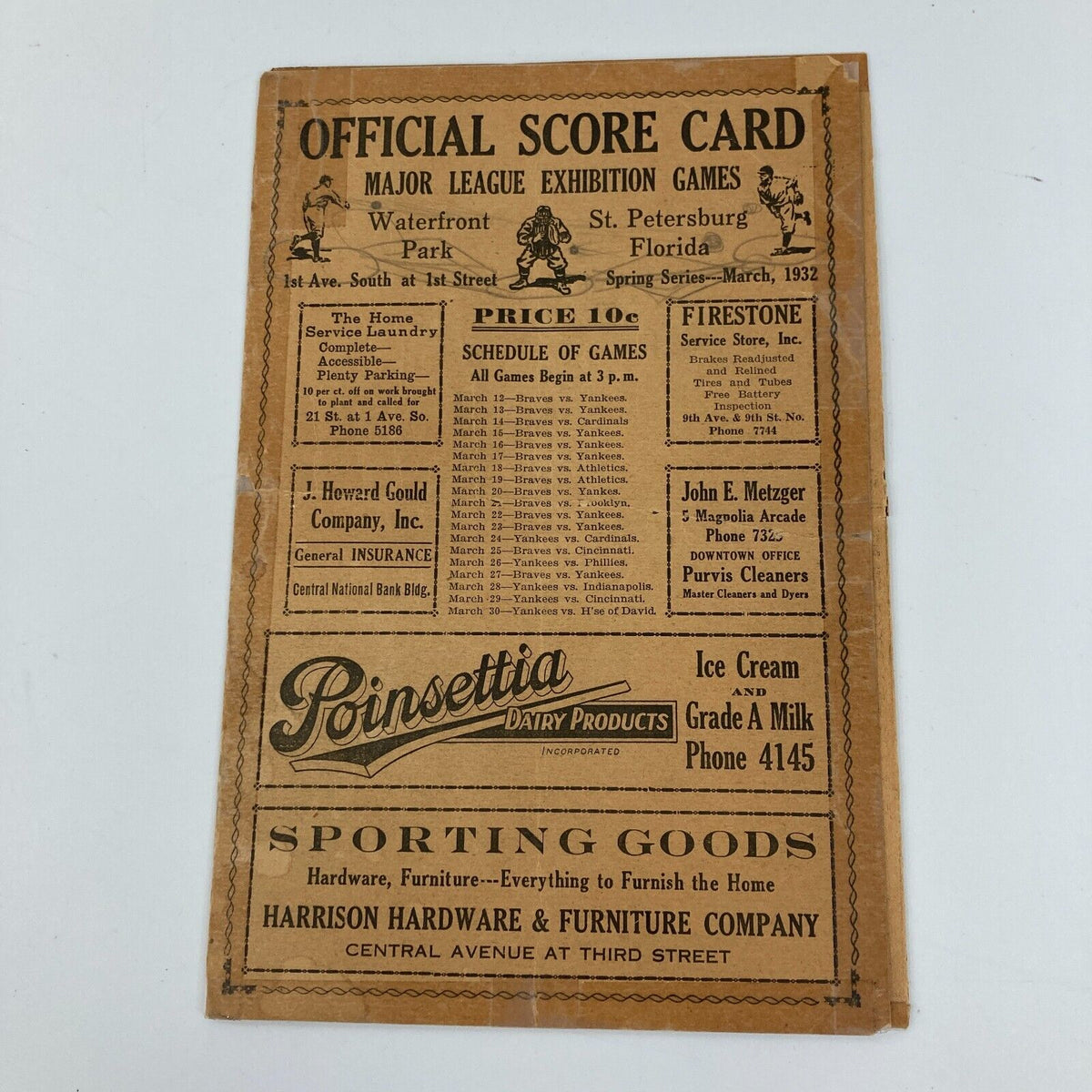This photograph, likely taken in a light box or on a copy stand, features a vintage baseball scorecard against a white background. The scorecard is made of thicker paper that has yellowed over time, giving it a sepia tone. At the top, it states "Official Scorecard," specifically for "Major League Exhibition Games," held at "Waterfront Park, St. Petersburg, Florida," during the "Spring Series, March 1932." Additional details mention the location at "First Ave. South at First Street." Decorative clip art-style drawings of baseball players adorn the upper section of the scorecard.

The scorecard includes a schedule of games, all beginning at 3 p.m., featuring teams like the Yankees, Braves, and Cincinnati. The price of the scorecard is marked as "10 cents." Alongside the schedule, various advertisements are displayed, such as:
- "Poinsettia Dairy Products," offering "Ice Cream" and "Grade A Milk," with a contact number, "Phone 4145."
- "Sporting Goods, Hardware, Furniture," provided by "Harrison Hardware and Furniture Company," located at "Central Avenue at 3rd Street."
- "Firestone Service Store."
- "Home Service Laundry."
- "J. Howard Gould Company, General Insurance."
- "Johnny Metzger, Purvis Cleaners."

The advertisements reflect the prominent businesses of that era, emphasizing the historical value of the scorecard. Overall, this vertical piece encapsulates both the sporting events and the commercial landscape of early 1930s St. Petersburg.